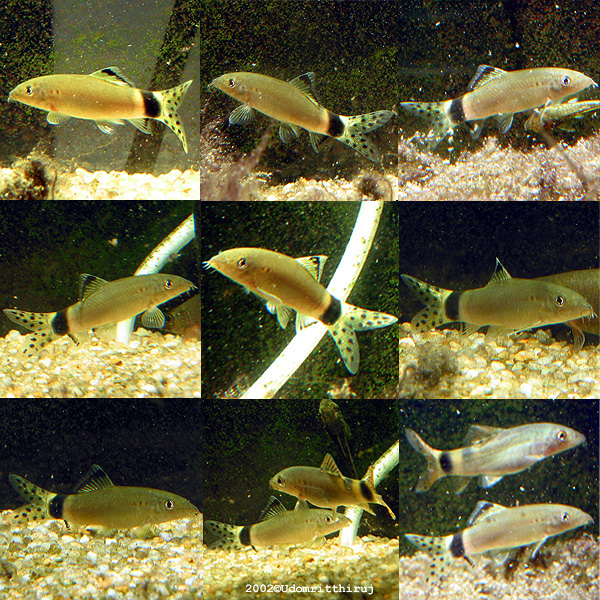This detailed color photograph showcases a series of nine individual square images, each capturing a close-up view of what appears to be the same small aquarium fish, or at least the same species, within the same tank. Arranged in a 3x3 grid, the fish is primarily brownish with hints of green, featuring a distinct black band around its tail, which transitions to a lighter, almost white color towards the tail end. The tail itself is green with black polka dots. 

In the first row, the left two images show a single fish facing left, while the right image has the fish facing right. In the middle row, the left image shows a fish looking right, accompanied by either a reflection or another fish looking left. The center image has one fish looking up and slightly left, and the right image includes two fish, with one facing right and the other's direction obscured. The bottom row's left image contains one fish facing right, the center image features two fish looking in different directions, and the rightmost image displays two fish, one above the other, both facing right.

The aquarium backdrop consists mostly of light-colored rocks such as white and yellow, with added visual interest from a lit tube visible in the leftmost and center images. A small piece of white text at the bottom, partially obscured by rocks, appears to read "2002 Copyright Udom Rithiruj," though it's difficult to discern clearly.

Overall, the fish, resembling a miniature shark with translucent and patterned fins along with eyes matching its grayish body, is shown swimming in various directions across a dark aquarium background sprinkled with tiny white specks, enhancing the visual texture of each frame.